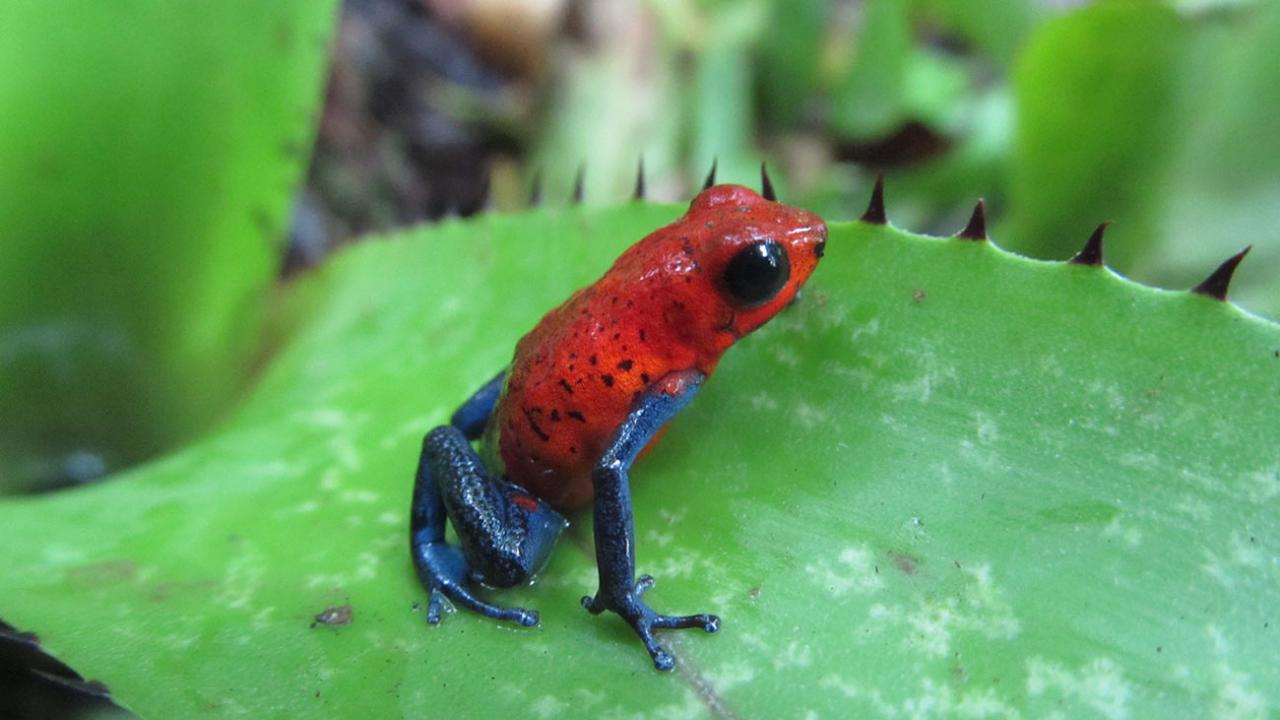The image captures a small, brightly colored poison dart frog perched on a wide, green cactus leaf adorned with thick, black, pointed spikes at its edges. The leaf itself is subtly speckled with faded white spots. The frog is in a crouched position, supported by its shiny blue legs and arms, while its body is vivid red, adorned with distinctive black dots. Its large, black eye with a small white reflective dot stands out prominently, giving it a striking appearance. The background of the photograph is a blur of greens and dark purples, suggesting other foliage but leaving the frog and its unique perch as the clear focus of the image.